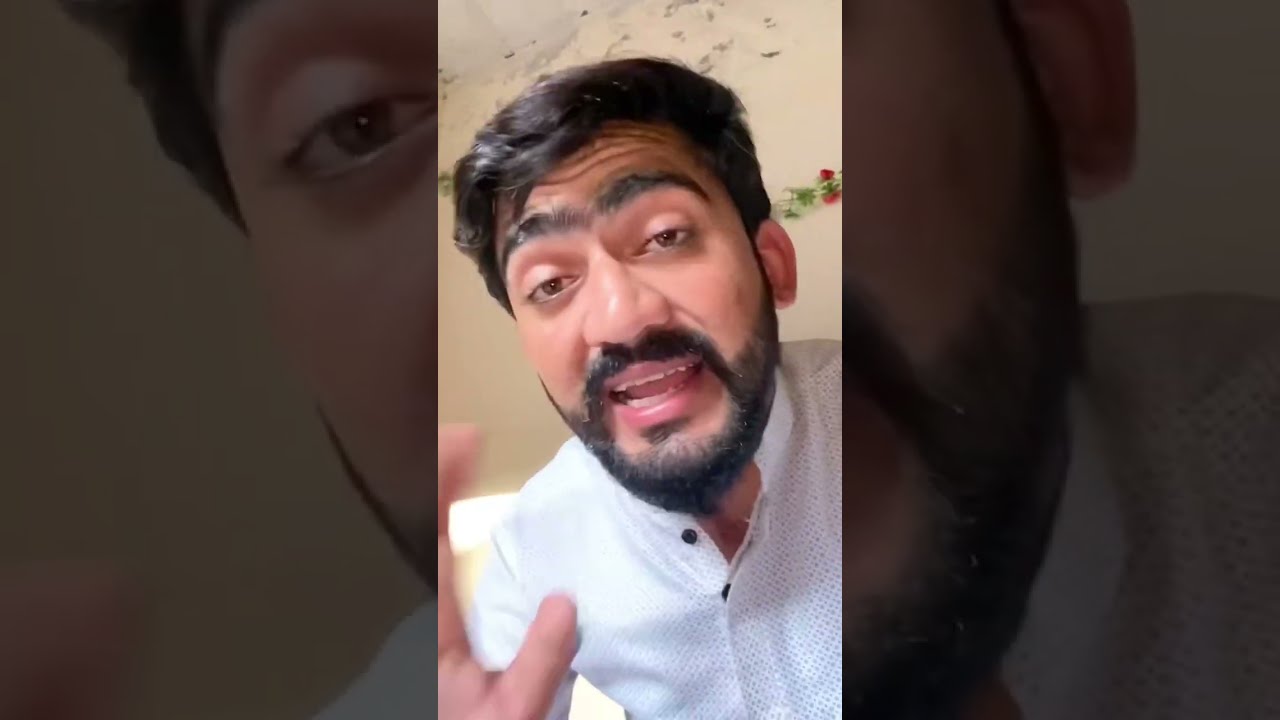The image depicts an up-close, full-color photograph of an Arabic male with dark complexion, thick black hair, and very bushy eyebrows forming a unibrow. His neatly trimmed, close-cut beard and mustache frame his face as he looks directly into the camera, his eyebrows raised and eyes engaged. The man is wearing a white button-up shirt, possibly with brocade detailing, and he's captured mid-speech, his hand gesturing in a way that appears slightly blurred due to motion. The composition of the image is unique, with the central panel displaying the man's face clearly, while identical side panels replicate this image, creating a layered effect. The background behind his head is plain and white, with some minor details such as small red and green flowers visible in one spot, although largely unnoticeable. The middle image appears overlaid against an even larger, more background-like version of the same image, creating a subtle, almost watermark-like effect.